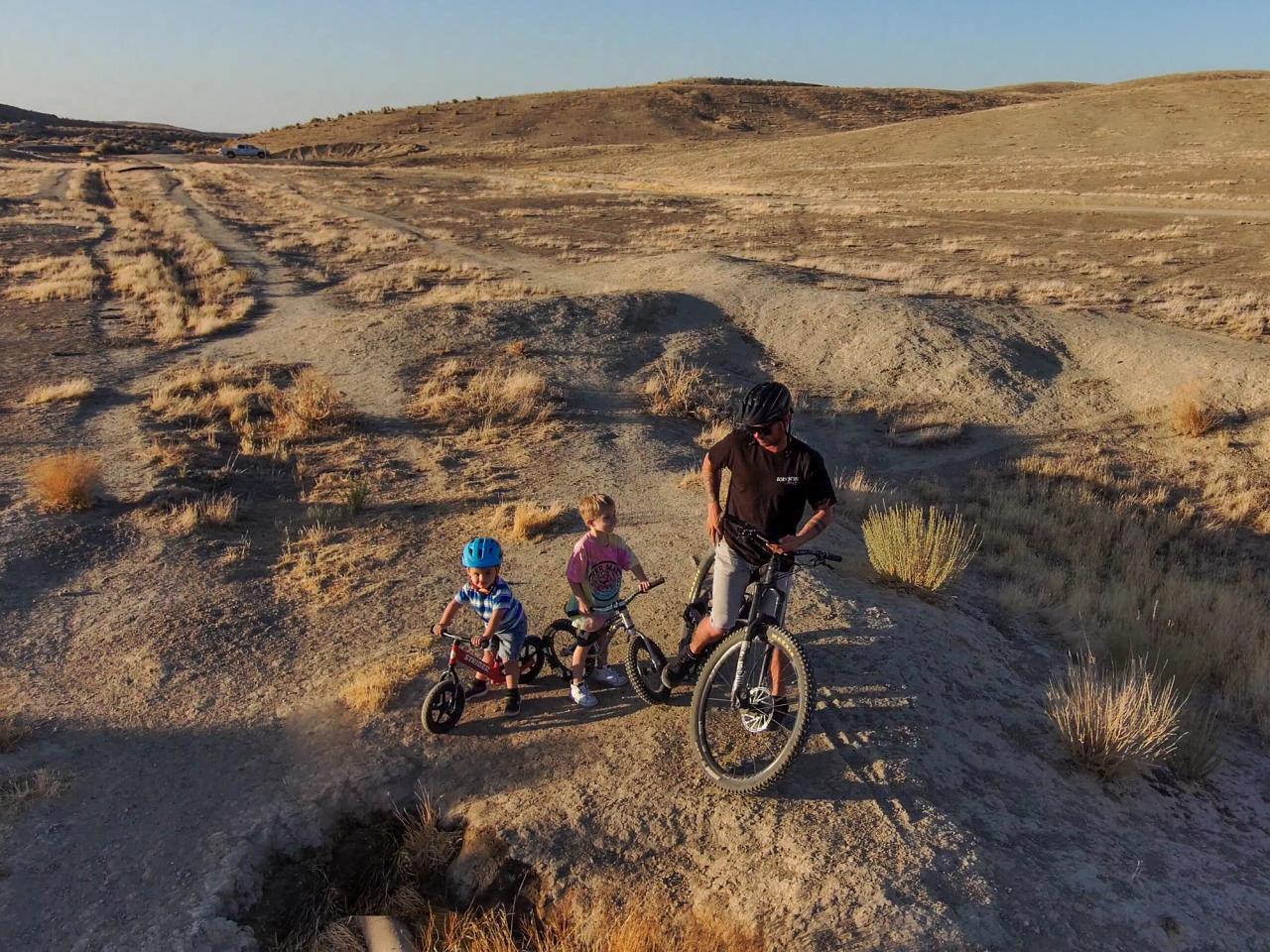The image depicts a vast, arid desert landscape with shades of brown, tan, and patches of dark black dirt, under a light blue sky that may suggest the late afternoon. In the distance, three main hills rise against the horizon, and an open-bed truck can be seen parked far away, possibly the starting point for the three individuals featured in the foreground. Up front, a father and his two young children are biking on a sandy trail. Both children ride small bicycles; the younger one sports a blue and white striped shirt, shorts, sneakers, and a light blue helmet while riding a red and white Strider bike. The older child is dressed in a pink shirt, shorts, and sneakers, holding their helmet rather than wearing it. The father, outfitted in a dark brown T-shirt and a black bike helmet, rides a larger bike. The barren landscape lacks any green vegetation, consisting solely of dirt and sporadic brown grass, indicative of a remote, popular biking spot in the wilderness.